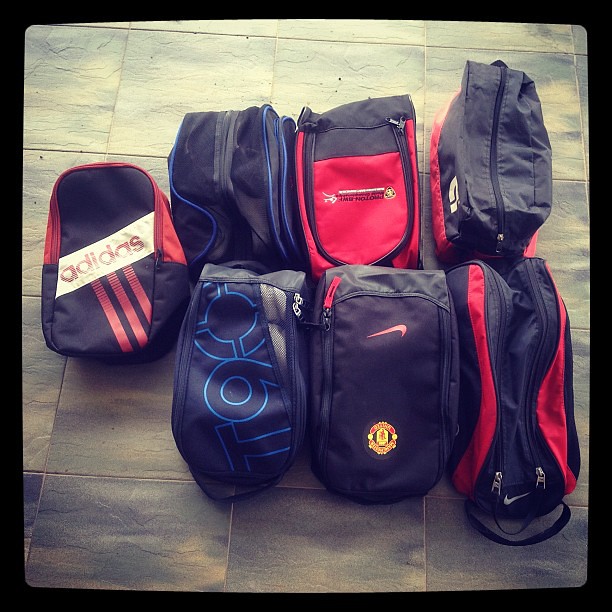The image is a detailed, organized display of seven athletic-style bags arranged on a grayish, textured tile floor. The bags, reminiscent of backpacks or duffel bags, are varied in color and brand. Six of them are positioned in two neat rows of three, while the seventh bag is set off to the left. The designs feature prominent branding, with some bags displaying the Nike swoosh and others the Adidas logo. A few bags have distinct text like "T90" and other logos, although some markings are illegible. The most visually notable details include the red, black, and white color combinations, along with some blue and light blue accents. One bag showcases a red and white diagonal stripe with red Adidas lettering, while another black bag features blue stripes in a "T90" formation. Each bag is equipped with zippers and various organizational features, indicative of the nylon and sports-specific design tailored for athletic utility.